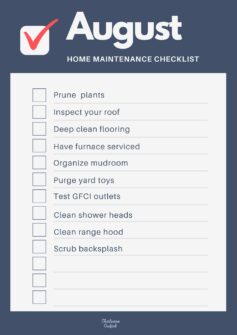The image features a "Home Maintenance Checklist" for August. Surrounding the checklist is a gray border. At the top, within the gray border, is a prominent checkbox with a red checkmark, next to which the month "August" is written in white letters. Below, the main content is situated inside a white box. Each maintenance task is prefaced by a checkbox, followed by the task description. The listed tasks include:

- Prune plants
- Inspect your roof
- Deep clean your floors
- Have the furnace serviced
- Organize your mud room
- Purge the yard toys
- Test the GFCI outlets
- Clean the shower heads
- Clean the range hood
- Scrub the backsplash

Towards the bottom of the checklist, three blank lines are provided, each with an accompanying checkbox, allowing for additional personalized tasks to be added.